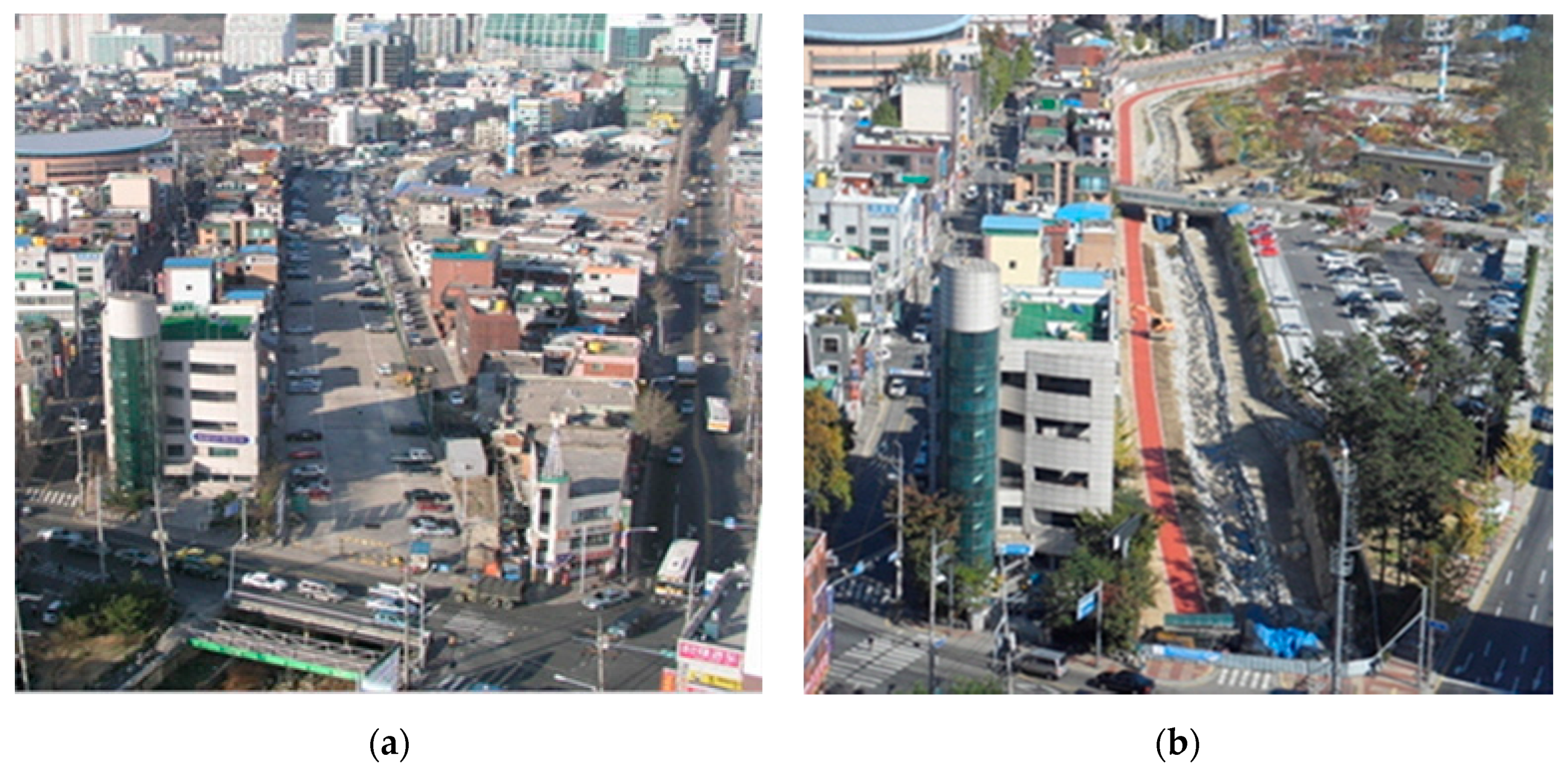The image consists of two side-by-side outdoor photos labeled A and B, both approximately square-shaped, capturing the same congested city from a similar angle but at different times. Photo A, on the left, shows busy streets with parking on each side and numerous cars. Tall buildings flank the streets with some skyscrapers visible in the background. A notable feature is a white high-rise building with a green and white tower. In contrast, photo B, on the right, appears to be a more zoomed-in, later version of the same scene. Some changes are evident in photo B: a canal with water and a walkway now runs through what was previously a road lined with cars. Additionally, a parking lot filled with vehicles has replaced some city buildings. The roads and infrastructure seem updated, featuring a reddish strip traversing its length. Consistent across both images is the prominent green-topped white building, underscoring the city's evolution over time.